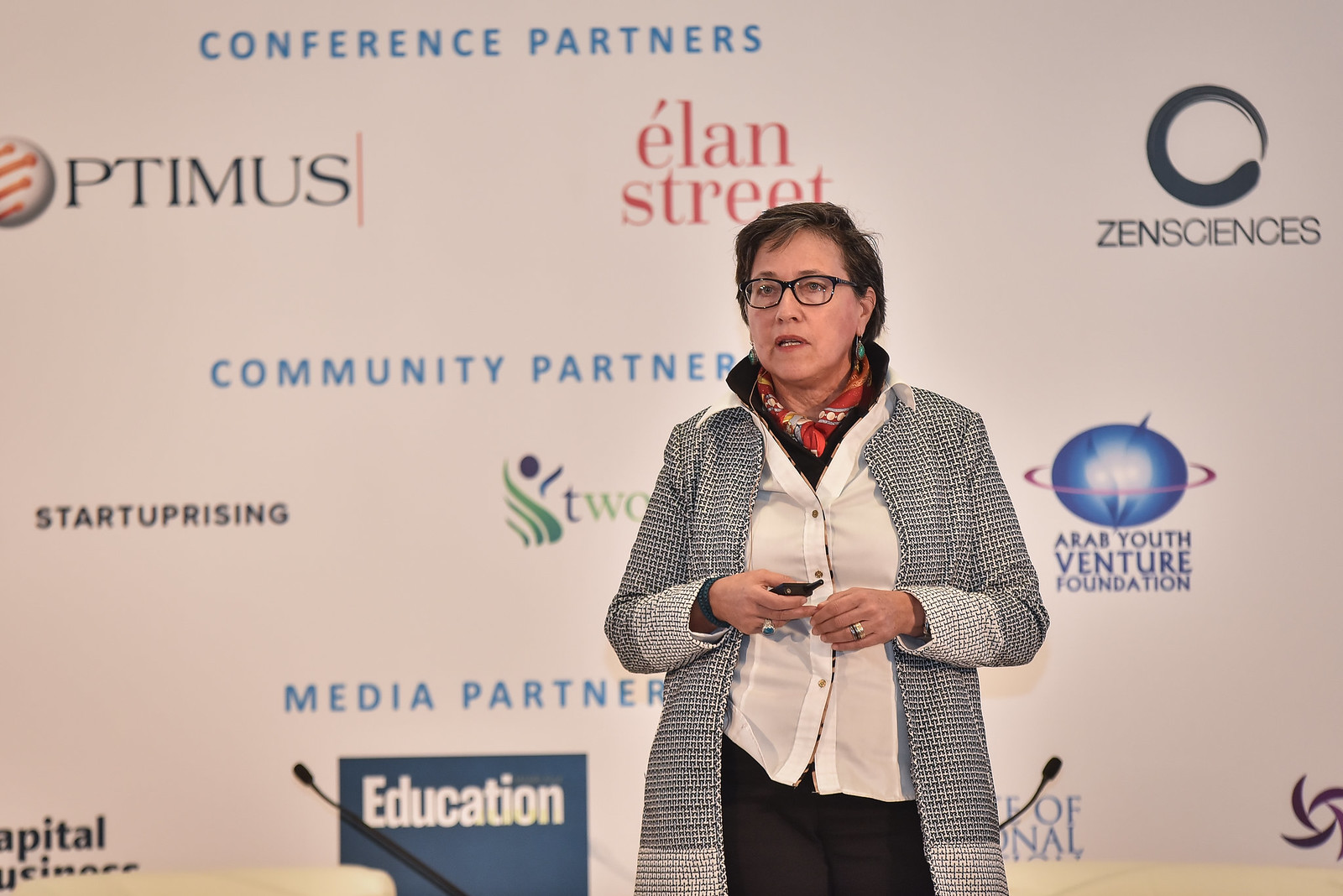A woman with short brown hair, wearing black-rimmed glasses, stands on a stage at what appears to be an exposition or conference. She is dressed in a white button-down shirt, black pants, a checkered black and white blazer, and a colorful scarf around her neck. Green earrings add a pop of color. She is speaking into multiple microphones placed in front of her, mid-speech. Behind her, a backdrop features various logos and text related to the conference. Visible names include "Conference Partners," "Optimus," "Elan Street," "Zen Sciences," "Community Partners," "Start Uprising," "Arab Youth Venture Foundation," and "Media Partners," although some of the signage is obscured by her presence. The backdrop is adorned with colors including black, white, green, gray, red, yellow, orange, blue, and purple, indicating a vibrant and diverse event.